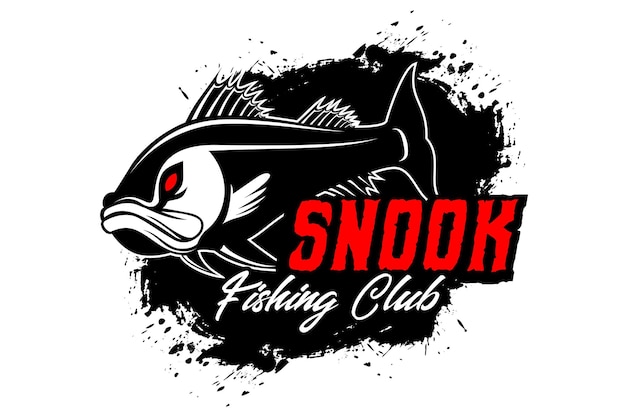The black and white image showcases an angry-looking fish, designed with a black body, white outlines and shading, and featuring a notably red eye. The fish's mouth is frowning and positioned towards the left side, while its tail extends towards the right. The backdrop is a white canvas, accentuated by a splatter of black paint, with speckles radiating outward. Prominently displayed on the image are large, bold, red block letters spelling "SNOOK" on the lower right side, and beneath it, in cursive white lettering, is the phrase "FISHING CLUB." The overall appearance is animated, with a clear and bright presentation, highlighting the stark contrasts and details effectively.